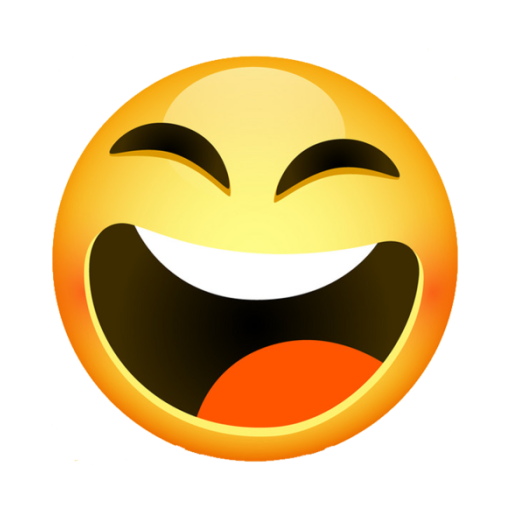The image features a large, detailed rendering of a laughing emoji set against a clean white background. Unlike typical emojis found on phones and social media, this one is notably bigger and more intricately shaded. It showcases a face with eyes shaped like upward-bent quarter moons, giving a sense of intense laughter. The eyes appear as black lines atop lighter yellow sections of the face. The mouth is open wide, revealing upper teeth and an orange tongue set against a background split by color: the upper part of the mouth is white, while the lower part is a darker orange-red shade, almost giving the impression of blushing cheeks. The emoji's design includes nuanced shading, with pockets of lighter yellow on the forehead and deeper orange-red tones around the mouth, adding depth and a sense of dimensionality.